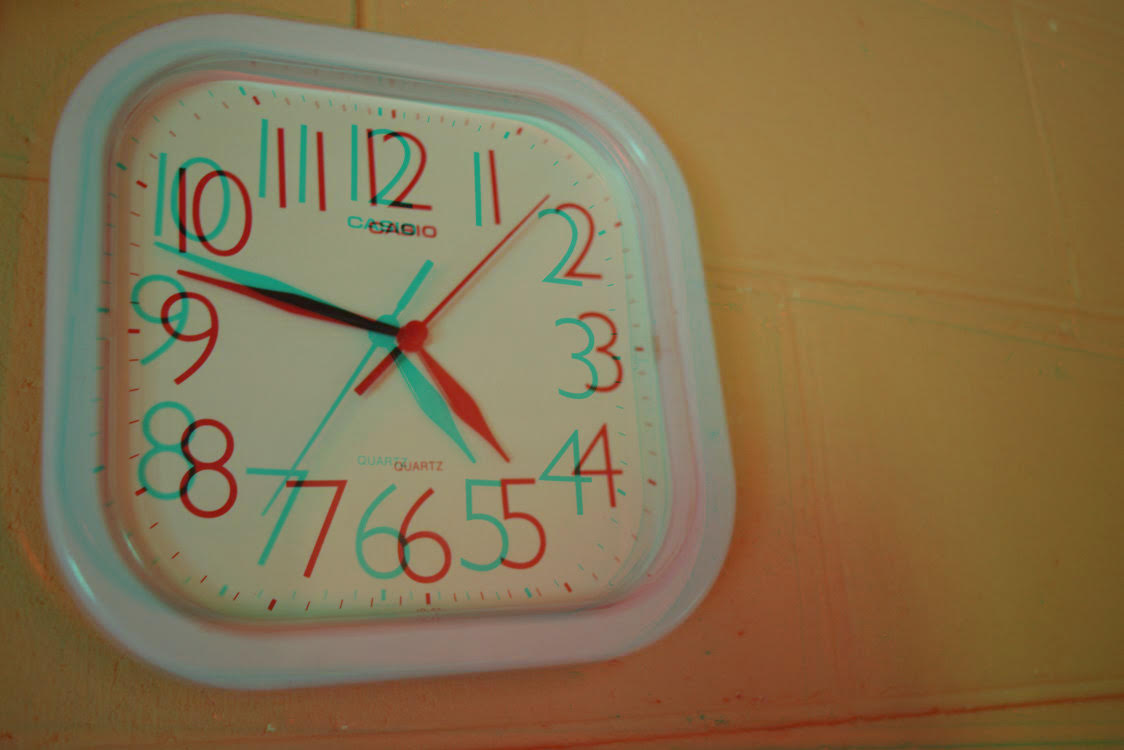The image features a square-shaped wall clock with rounded, curvy corners, mounted on a mustard-yellow painted cinder block wall. The clock's white plastic frame encases a unique design where each numeral from 1 to 12 is duplicated, creating an optical illusion. One set of numbers is red, and the other is teal blue, giving the appearance of shadows or a 3D effect which makes the clock seem blurry or out of focus. The clock has three red hands: the long minute hand is positioned between 9 and 10, the short hour hand points to 5, and the thin second hand is between 1 and 2. Just below the number 12, the word "cashier" is printed. This intricate design makes the clock look like it is shaking or moving, adding to the visual complexity.